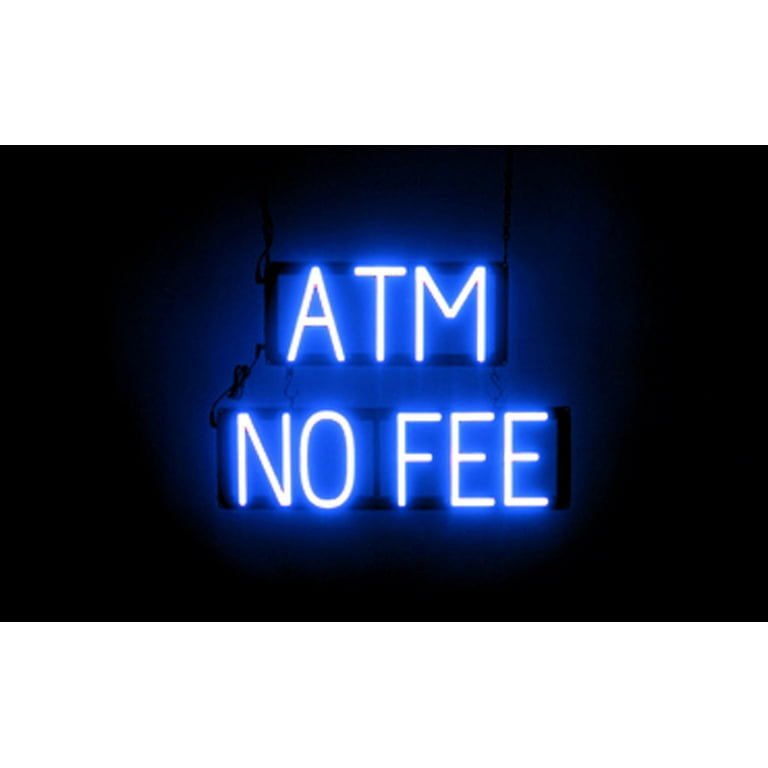The image depicts a photograph of a neon sign centered against a completely black background. The sign consists of two distinct parts. The upper section has the word "ATM" in bright white capital letters, surrounded by a bluish glow that creates a striking contrast with the dark background. Below this, connected by a visible black wire, is a second part with the words "NO FEE" also in white capital letters, similarly illuminated by a blue hue. The overall structure of the sign is rectangular with a dark border, and the glowing elements suggest it is likely positioned to guide users to an automatic teller machine, emphasizing the absence of usage fees.